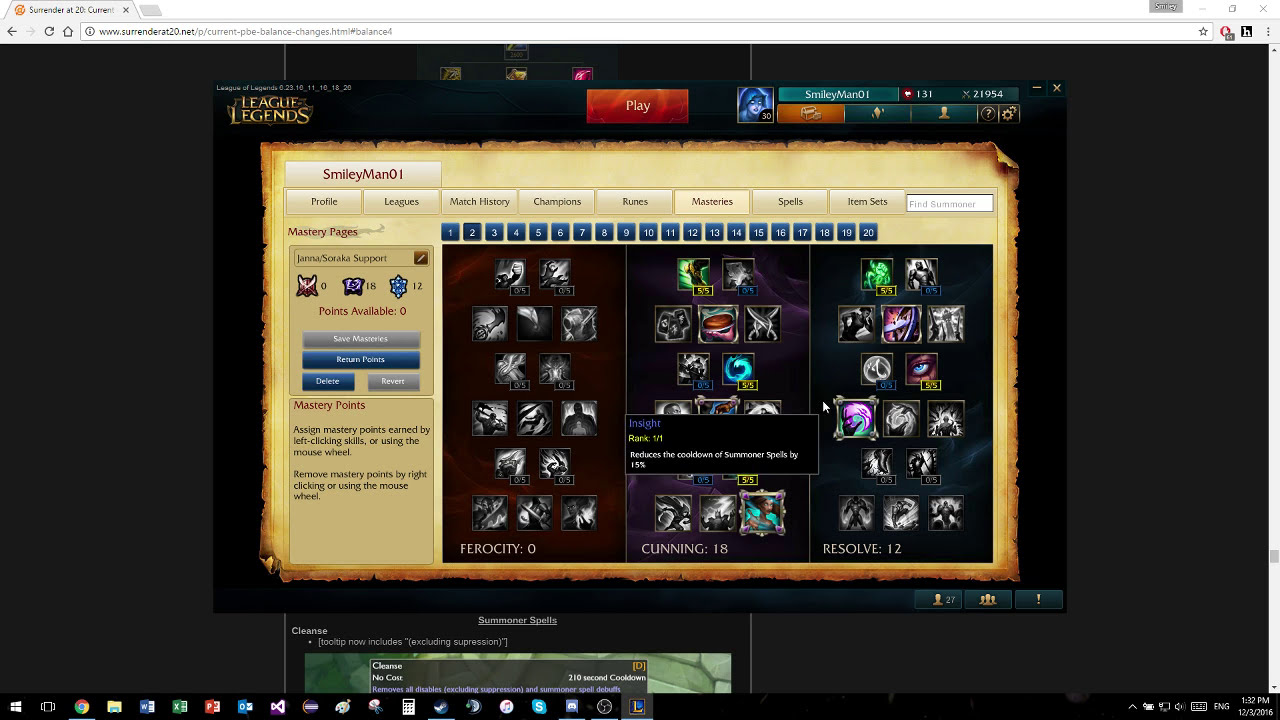This image is a detailed screenshot captured from a Windows computer, showcasing a web browser that is open to what appears to be a game dashboard for "League of Legends." The recognizable League of Legends logo is visible in the top-left corner, although slightly unclear. The screenshot includes the Windows taskbar at the bottom, featuring icons for various software applications like Google Chrome, My Documents, and Microsoft Excel, confirming that it's taken from a desktop environment.

The main section of the browser displays a comprehensive game interface divided into four sections. The player, identified by the username smileyman01, has options labeled as Profile, Leagues, Match History, Champions, Runes, Mastery, Spells, and Item Sets. Noteworthy elements within these sections include mastery features such as points available, save points, and return points, along with graphical representations of different mastery branches: Ferocity, Cunning, and Resolve.

Prominently positioned in the center of the interface is a large red button labeled "Play," indicating that this is the game's introductory screen or dashboard from which gameplay can commence. The screenshot is rich with various colors including gray, black, yellow, red, purple, green, pink, and blue, all contributing to the vibrant and intricate design typical of an online game dashboard.